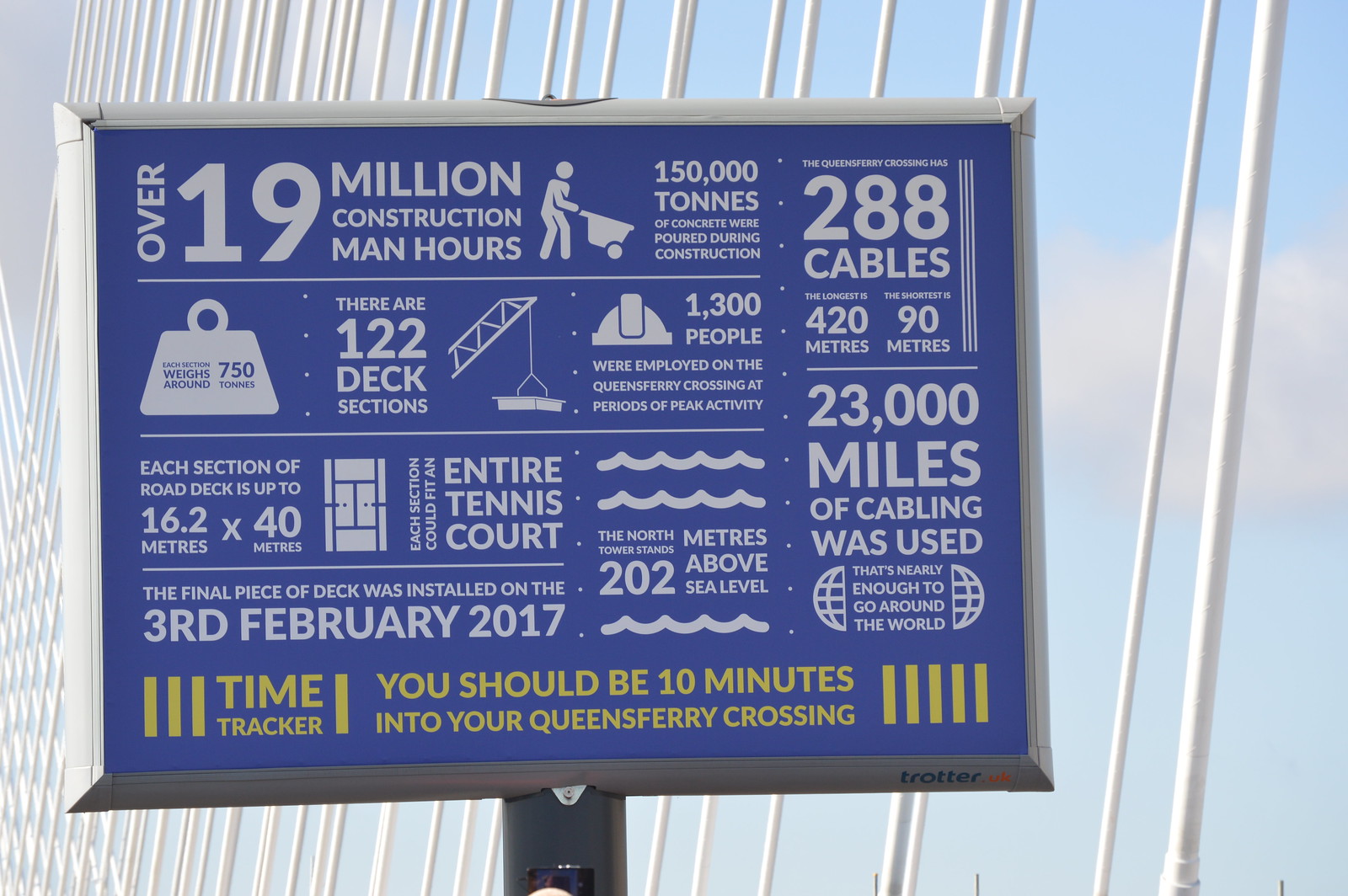This detailed photograph captures an outdoor setting on a beautiful day with a striking blue sky dotted with some clouds. Dominating the image is a large blue sign with a gray metal frame, mounted on a metal pole, though only the top part of the pole is visible due to cropping. The sign, positioned centrally, is flush with intricate details and compelling visuals that capture the monumental effort behind the construction of the Queensferry Crossing. The sign features predominantly white text, interspersed with numbers and facts in a structured layout. 

Prominently, it states "Over 19 million construction man hours" at the top left, bordered by white lines separating different sections of information. Detailed statistics include "150,000 tons of concrete were poured during construction," "288 cables, with the longest measuring 420 meters and the shortest 90 meters," and "93,000 miles of cabling was used"—enough to nearly encircle the globe. It also highlights that "1,300 people were employed at peak activity" and there are "122 deck sections."

Adding visual interest, the sign is adorned with various graphics, like a stick figure with a wheelbarrow and a construction crane lowering a metal piece, next to the text. The bottom of the sign features yellow text, proclaiming "Trotter" on the left alongside a vertical yellow bar, and reminding viewers, "you should be 10 minutes into your Queensferry Crossing," flanked by five vertical yellow lines on the right.

In the background, white beams—inferred to be parts of a bridge—stretch upwards, enhancing the construction theme of the scene. The overall color palette includes blue, white, gray, yellow, and touches of black, juxtaposing the detailed information with an aesthetically pleasing and informative design.